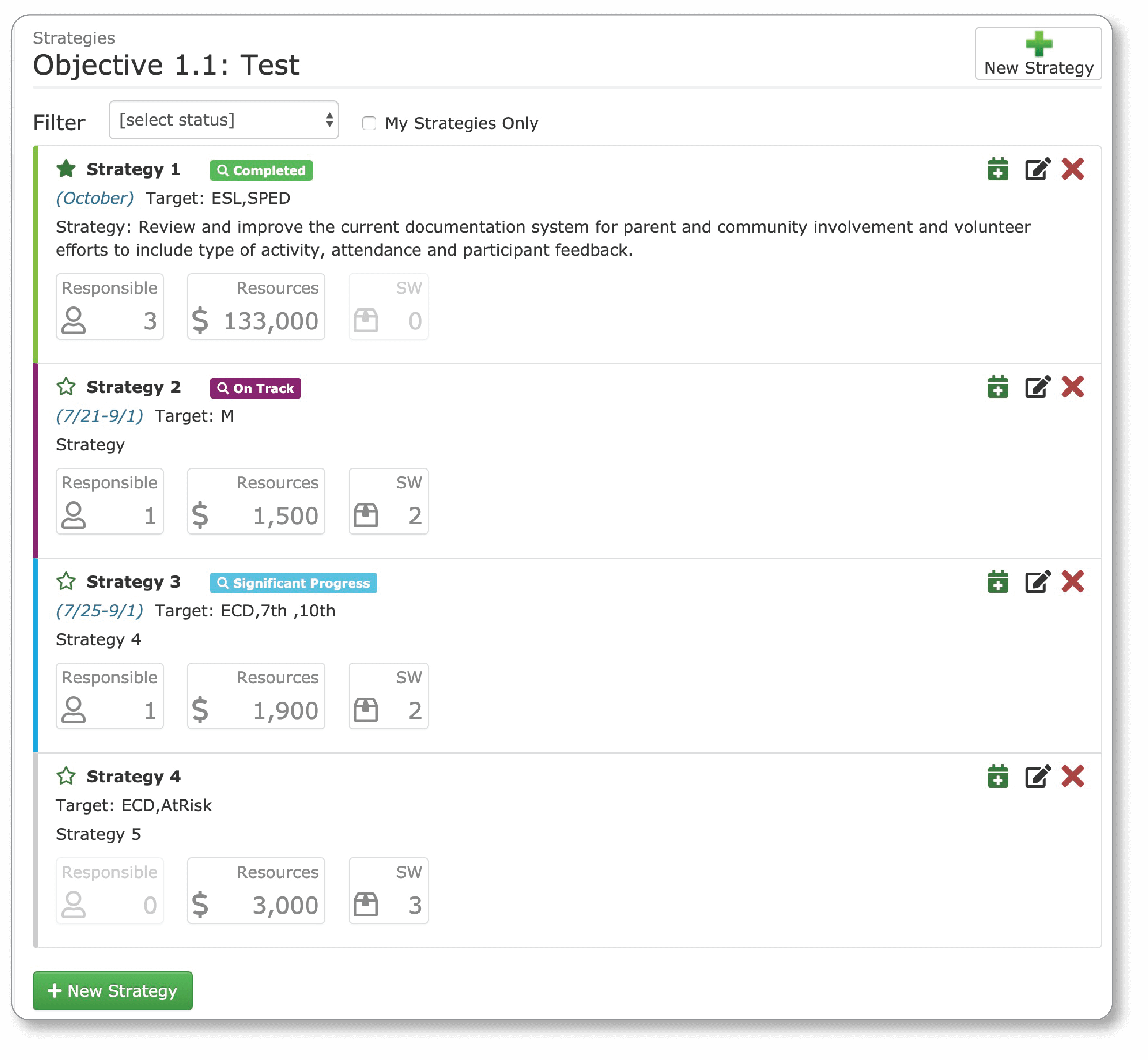The image displays a detailed form titled "Strategies" at the top. Immediately below this title, it lists "Objective 1.1: Test". To the right side, there is a green plus icon, and beneath that, it says "New Strategies". The form includes a section for filtering options, labeled "Select Status: My Strategies Only".

A section labeled "Strategy One" is marked with a green star, indicating that it is completed. The detailed description for Strategy One involves reviewing and improving the current documentation system for parent and community involvement and volunteer efforts, including documenting the type of activity, attendance, and participant feedback. This strategy has three responsible individuals and a budget of $133,000 allocated for resources.

The subsequent strategies are listed as follows:
- Strategy Two: Marked as "On Track", specifying one responsible person and $1,500 in resources.
- Strategy Three: Targets "FCD, 7th, 10th", with one responsible person and resources amounting to $1,900.
- Strategy Four: Focuses on "ECD at risk" with an allocation of $3,000 in resources.
  
At the bottom of the form is another green button labeled “+ New Strategy,” which presumably allows users to add additional strategies.

The layout is organized and provides clear information about each strategy's status, the responsible parties, and resource allocation.